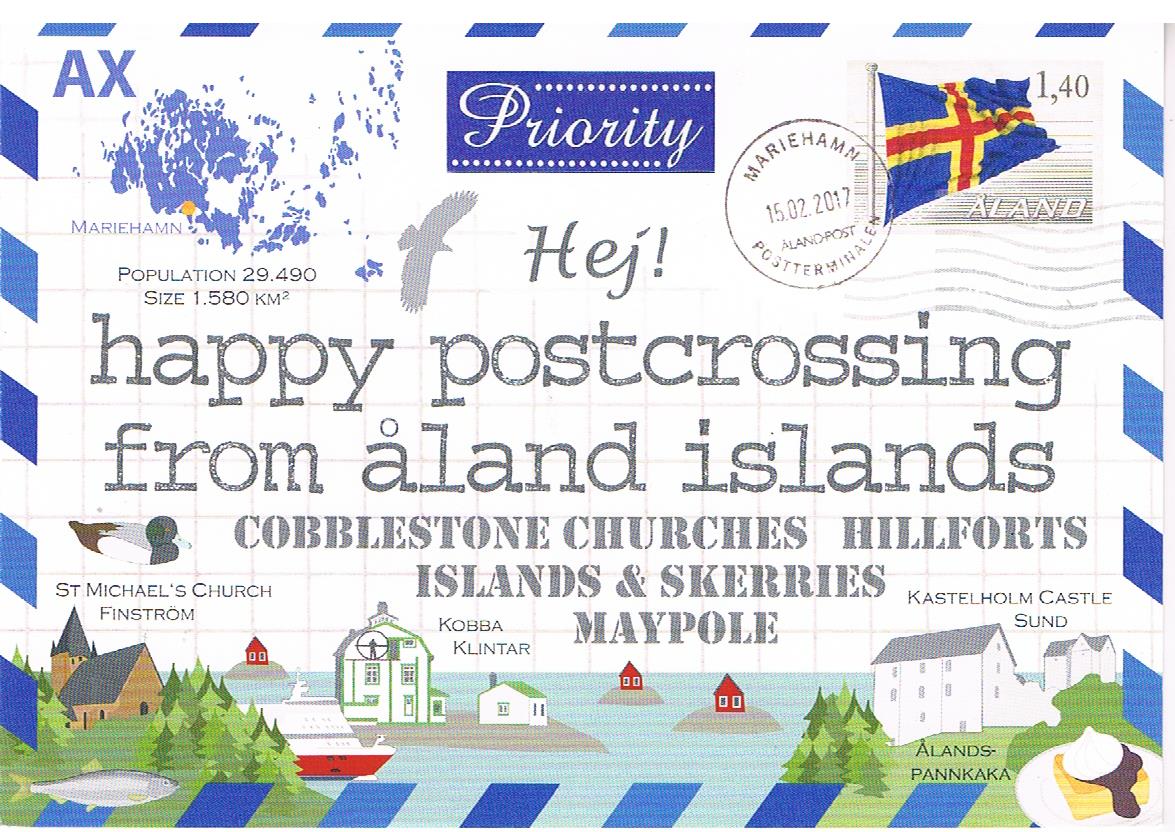The postcard from Maraheim, titled "Priority - Maraheim, 1502 - 2017," features a wealth of detailed information and imagery. Situated in the top left corner, it states "AX, Maraheim, Population: 29,490, Size: 1.580 km²." The top right corner displays the numerical code "1,4 0" alongside the flag of Olland—a blue background adorned with a white and yellow cross at its center. 

Central to the postcard's theme is the message "Happy Posts, Crossing from Olland Island," highlighting notable attractions such as cobblestone churches, hillforts, islands, and skerries, underlined by "Maraheim." Text in the middle indicates "Priority, Maraheim 1502 2017, Poster with Allen."

Detailed captions are placed around the postcard identifying various landmarks and sights: St. Michael's Church in Finstrum occupies the bottom left corner, with Cova Clintar noted just below it. To the right, there are mentions of Castleholm, Castle Sund, and Allen's Penkaka, showcasing the region's rich heritage.

The images themselves depict a variety of sceneries and elements characteristic of Maraheim: picturesque churches, lush trees, tranquil waters, a fish, and a delectable dessert featured at the bottom of the postcard.